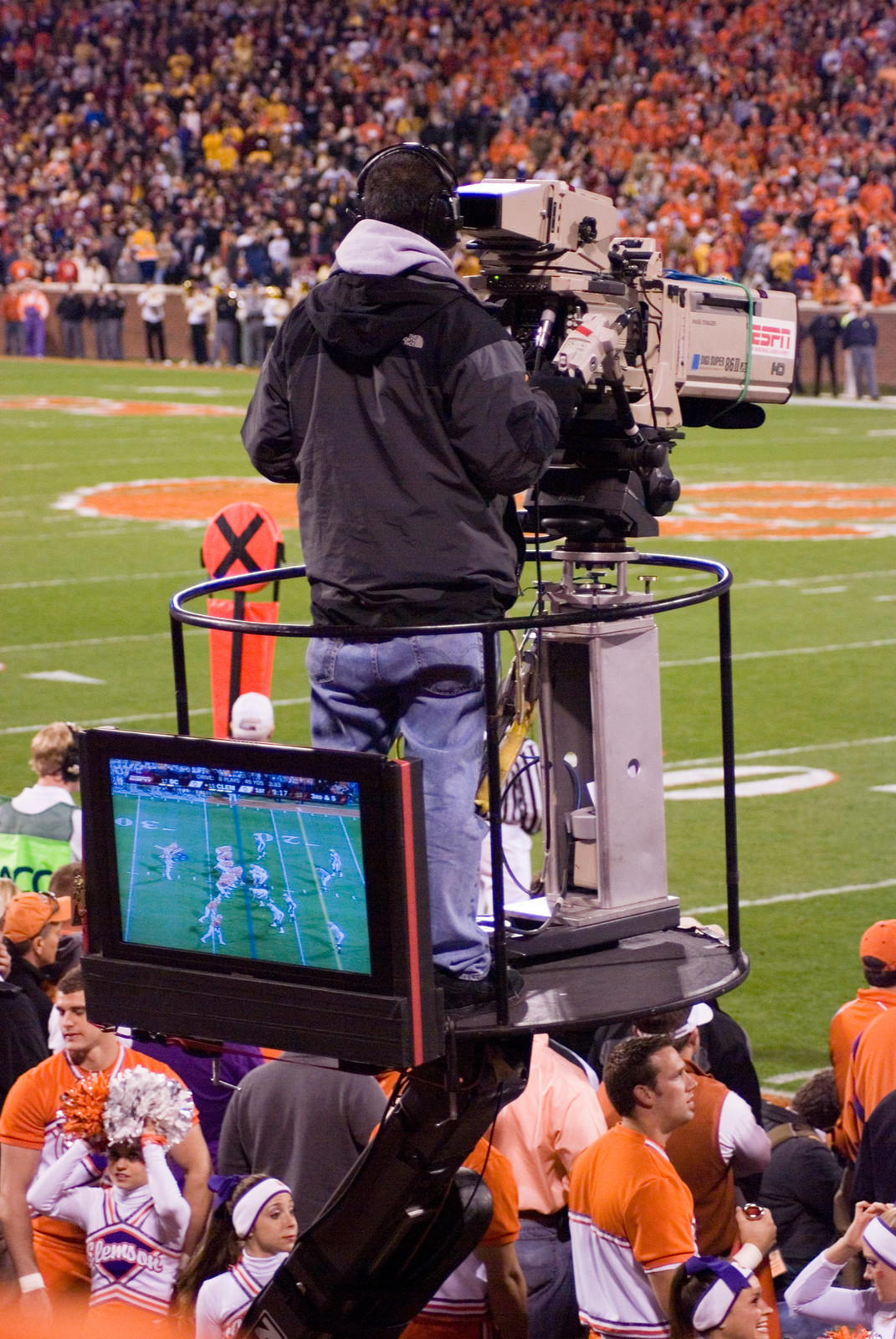A beautifully detailed photograph captures a dedicated cameraman at a football game, skillfully operating a large, mounted ESPN camera from a circular elevated platform. The cameraman, dressed in a long-sleeved black jacket, loose blue jeans, and black headphones, stands with his back to the viewer, intently focused on the action. His platform, surrounded by a guardrail, extends out over a crowd in the stadium below. Positioned at eye level, an LCD screen behind him displays a live feed of the game, revealing football players from opposing teams crouched and ready for play. Spectators fill the stands in the background, predominantly dressed in vibrant orange, which appears to be the home team color. The field, vividly green with white lines and orange markings, also features scattered cheerleaders in white uniforms with pom-poms, enhancing the dynamic, lively atmosphere.